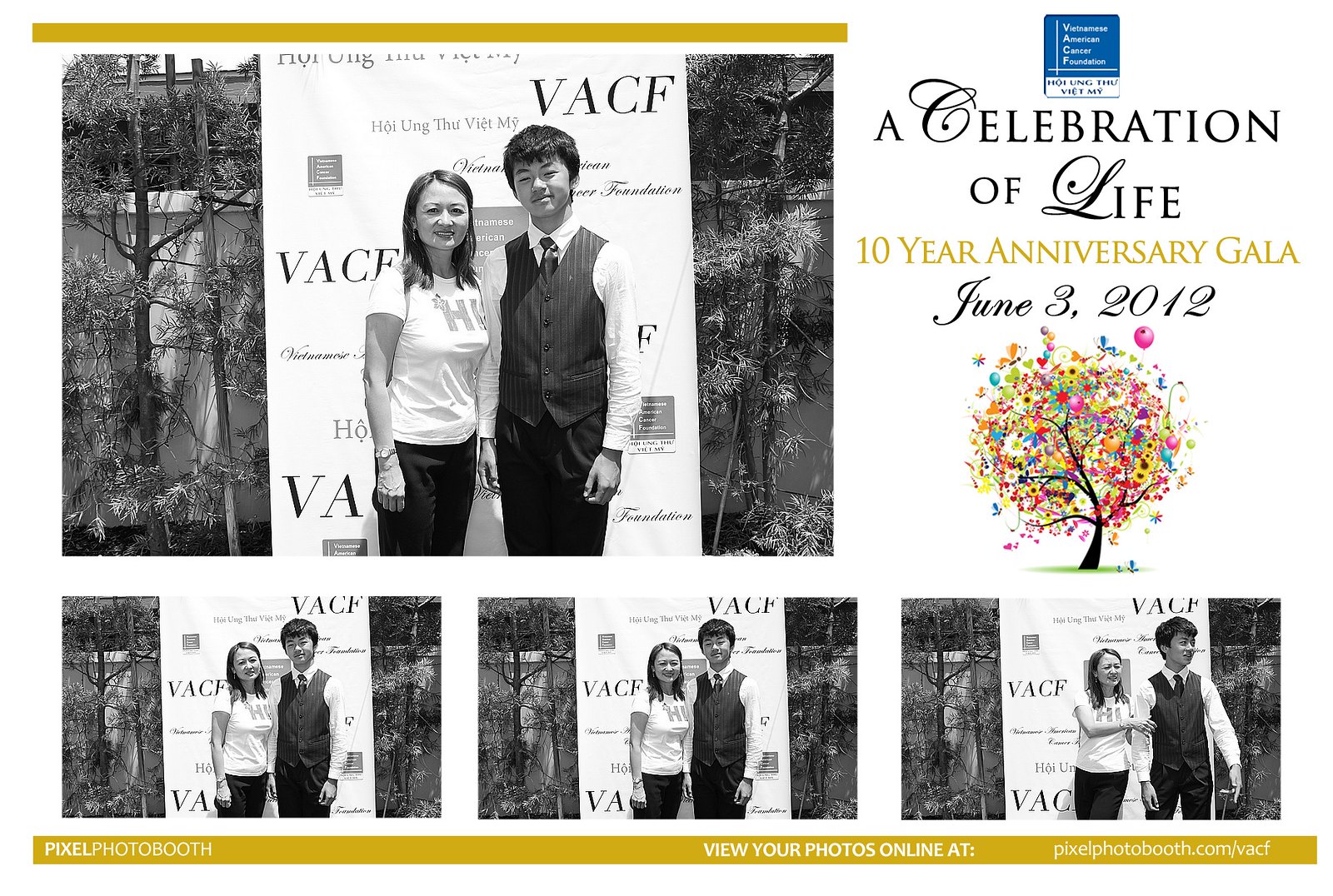The advertisement image prominently features the text "A Celebration of Life, 10 Year Anniversary Gala, June 3, 2012" at the top right corner, accompanied by a vibrant graphic of a tree with multicolored leaves. Below this text is a photo montage featuring an Asian boy and an Asian girl standing in front of a banner that reads "VACF." The main image is repeated three times along the bottom row, showing the couple in slightly different poses and hand movements, always smiling. To the left of the repeated photos, the backdrop includes trees against a white wall, indicating an outdoor setting. At the bottom of the ad, a long horizontal bar displays the text "Pixel Photo Booth" on the left, with "View your photos online at" in the center, and the website "pixelphotobooth.com" on the right in a clean, white font.